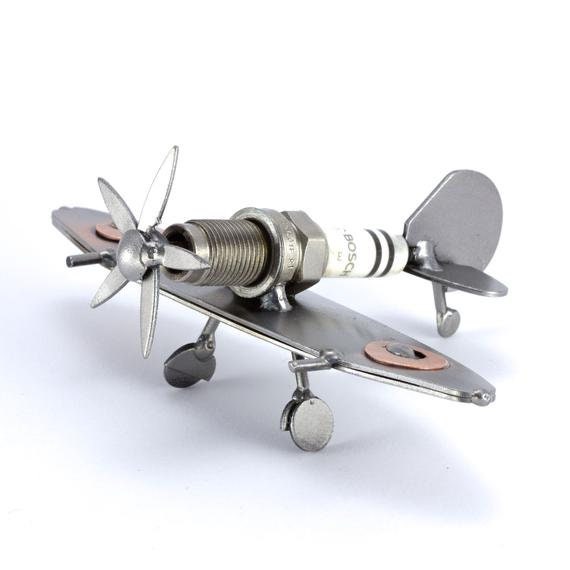The image showcases a meticulously crafted metal sculpture of a small propeller airplane, made from various everyday tools and metal items. The airplane's propeller is prominently featured at the nose, with five intricately fashioned blades. It rests on three wheels: two positioned under the main wings and one smaller wheel at the tail. The complex assembly includes screws, pipes, and welded joints, with recognizable brand names faintly visible on some components. Among the various tools used, a spark plug forms the main body, with its screw end facing forward, where the propeller is attached. The wings display small metal pins, possibly representing machine guns, suggesting that the plane might be modeled after a World War I aircraft. The background of the image features a sharp division with a blue section on the left transitioning to a predominantly white space, creating a distinct shadow under the plane. The entire piece exudes a high level of craftsmanship, appearing almost like a photograph but rendered with a quality that suggests it may be computer-generated or digitally enhanced. The plane is set diagonally, enhancing the dynamic aesthetic of the sculpture, and reflects the artist's remarkable talent in transforming mundane materials into detailed, evocative artwork.